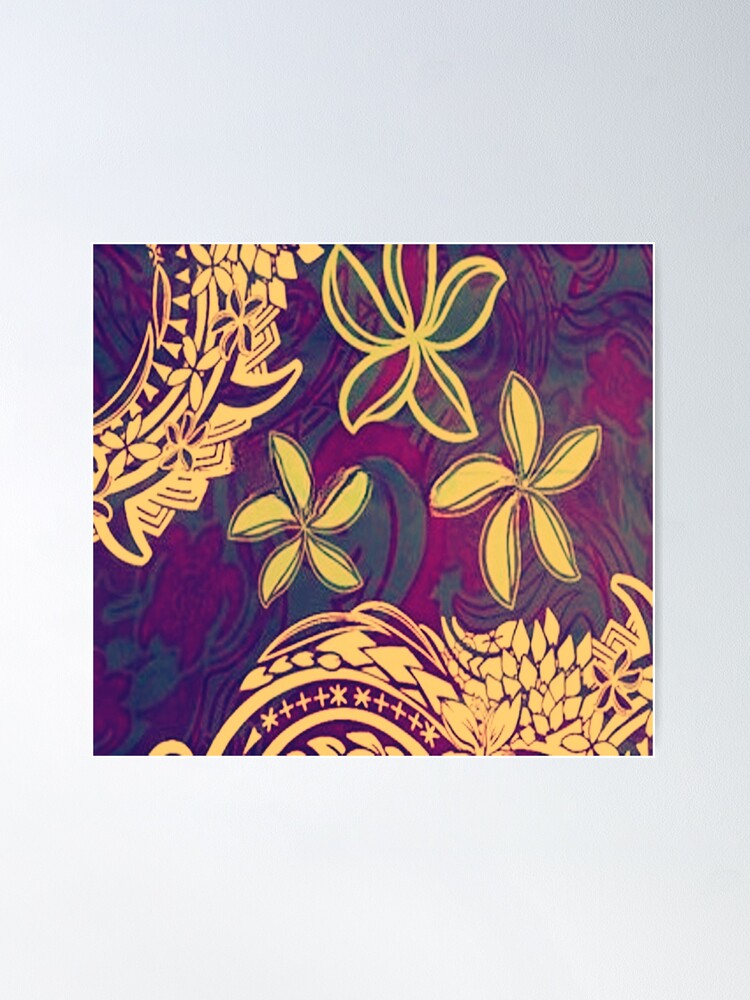This photograph captures a vibrant piece of art displayed against a perfectly smooth, light gray wall, giving an almost photoshopped appearance to the background. The central focus of the artwork features three bright yellow flowers, each adorned with five petals radiating outwards. Enhancing the floral composition are intricate mandala-like patterns located in the top left corner and the bottom right corner. 

The mandala in the top left corner is characterized by larger circles that form a tube-like structure, allowing the gray background to peek through. Conversely, the mandala in the bottom right corner is more expansive, occupying nearly two-thirds of the lower section of the image. These mandalas are rendered in varying shades of burgundy and dark green, adding depth and contrast to the overall piece. The combination of vivid flowers and geometric patterns creates a rich, dynamic visual experience.